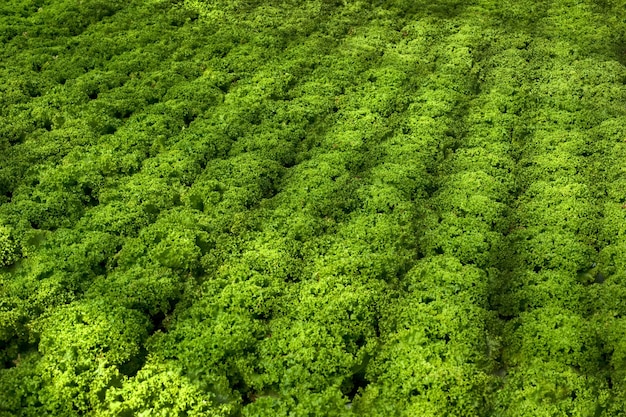This aerial photograph captures an expansive field of trees planted in uniform, closely spaced rows, their bright green foliage forming a lush, textured carpet that dominates the landscape. Each row is neatly defined, yet the overlapping leaves create a continuous, vibrant sea of greenery. The bright green shades vary, enhanced by patches of sunlight and shadows, particularly noticeable in the left lower quadrant. The repeated pattern of the foliage, with lighter and darker greens, adds depth and brilliance to the scene. The detailed texture of the leaves is distinctly visible, emphasizing the meticulous arrangement of this agricultural landscape.